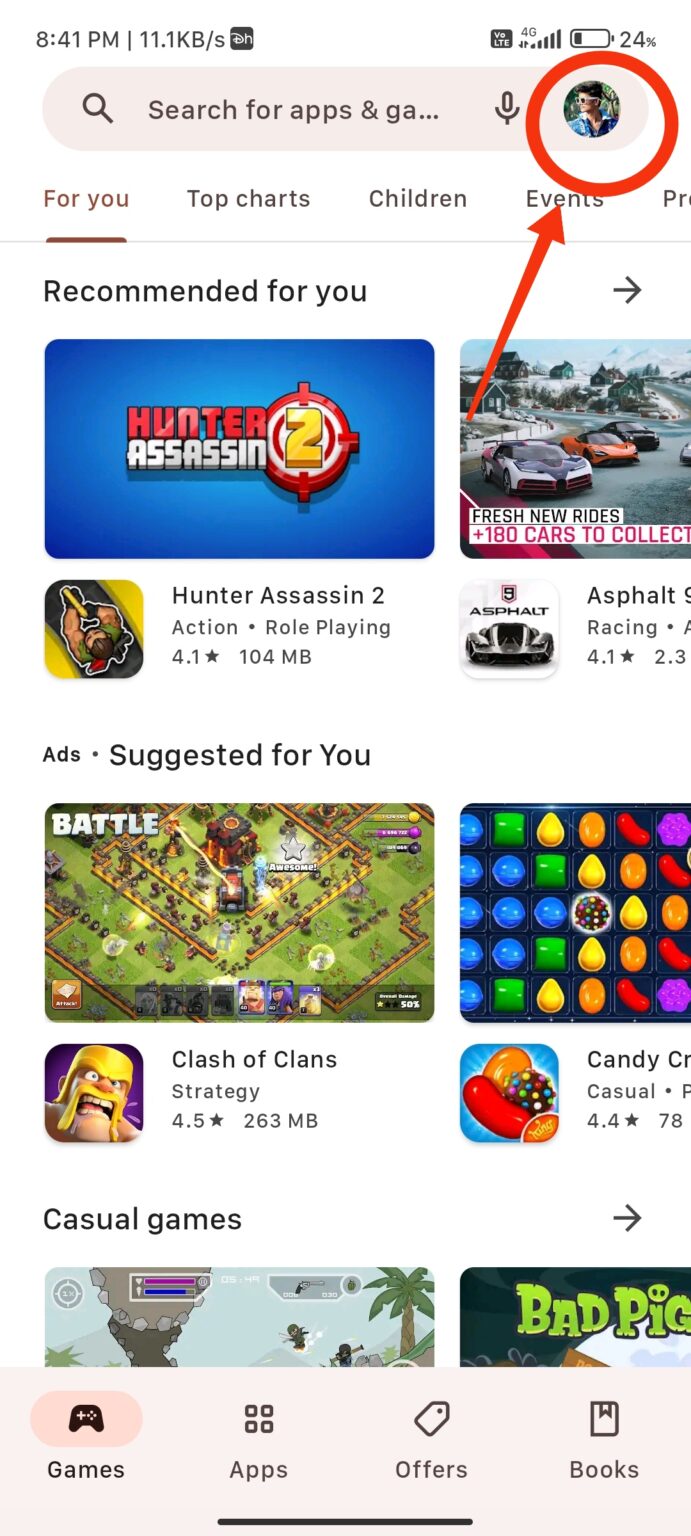Screenshot from a Smartphone Displaying Various Details:

The screenshot showcases a smartphone interface. In the top left corner, the time is displayed as 8:41 PM alongside a data transfer rate of 11.1 KB per second. The signal strength indicator shows four bars, and the battery level is critically low at 24%.

Below these indicators is a search bar that reads "Search for apps and games," with a circular profile picture on the right. The profile picture features a person wearing a blue garment and is highlighted by a red circle and a red arrow pointing towards it.

Under the search bar, a menu displays several options: "For you," "Top charts," "Children," and "Events," with a light-colored line beneath them. The section is labeled "Recommended for you," featuring a blue box with a red and white target and a gold number "2" within it. This box advertises the game "Hunter Assassin 2" in bold red and white capital letters.

The details of the game are listed as follows: "Hunter Assassin 2," categorized under "Action" and "Role Playing," rated 4.1 stars, and requiring 104 MB of storage. Below this, a section labeled "Ads suggested for you" appears, including a visual of a battlefield from above, accompanied by a green graph and several small icons.